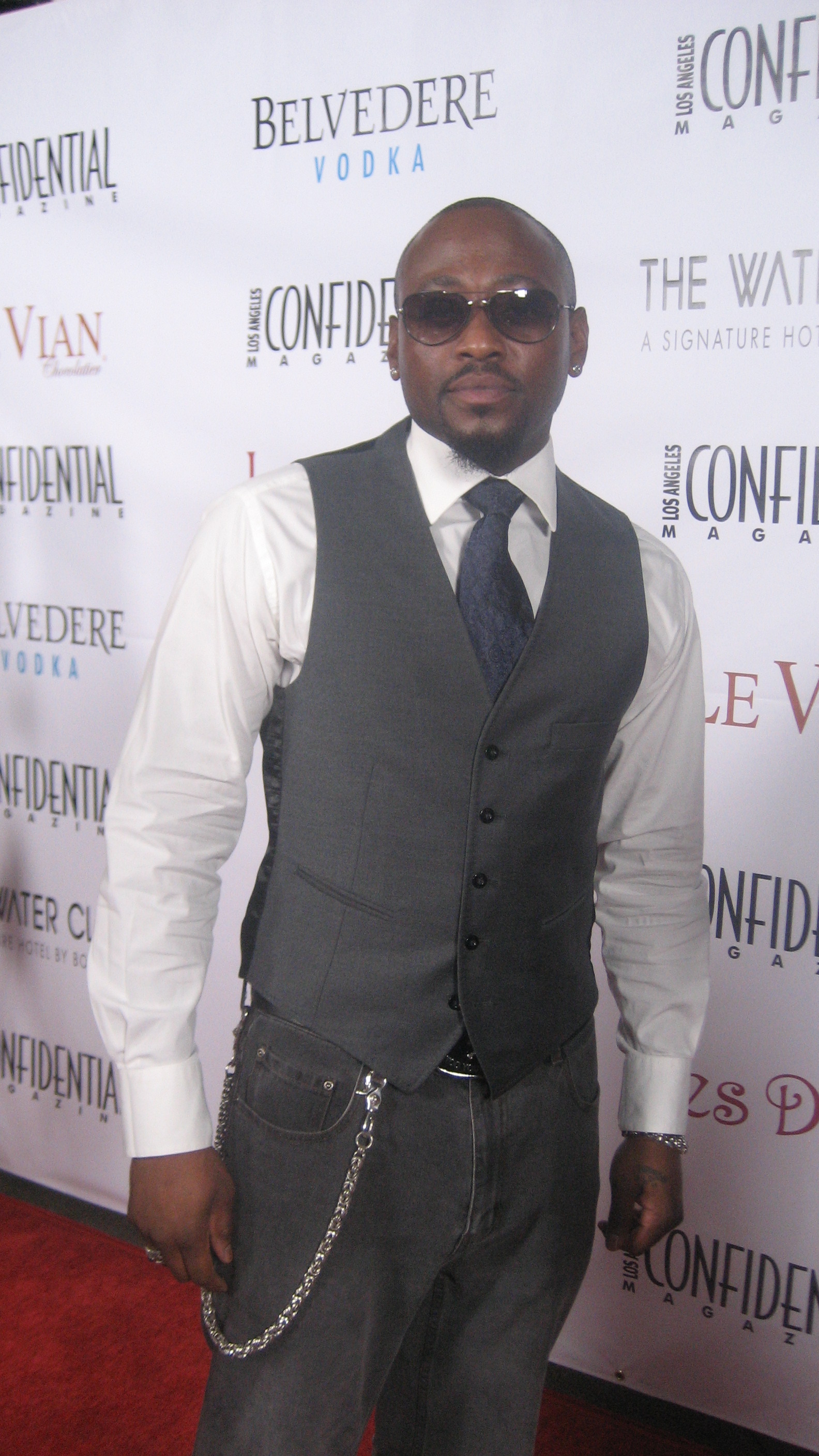The photograph captures a stylish black man, identified as Marlon, posing on a dark red carpet at a convention. Marlon, who has very little hair and a black goatee, is featuring aviator sunglasses with a tinted glass. He is dressed in a white collared shirt paired with a blue tie and layered with a dark grey vest. His ensemble also includes dark grey jeans, accentuated by a hook chain running from the front belt loop to the back. Marlon stands at a slight angle, with his right shoulder raised and his left shoulder lowered, his arms resting naturally by his sides. The backdrop is a large white banner featuring several logos, prominently displaying 'Belvedere Vodka' in black and blue font, and 'confidential' partially visible in black. The white banner's design also includes repeated logos arranged in a grid format, adding to the visual interest of the photograph.